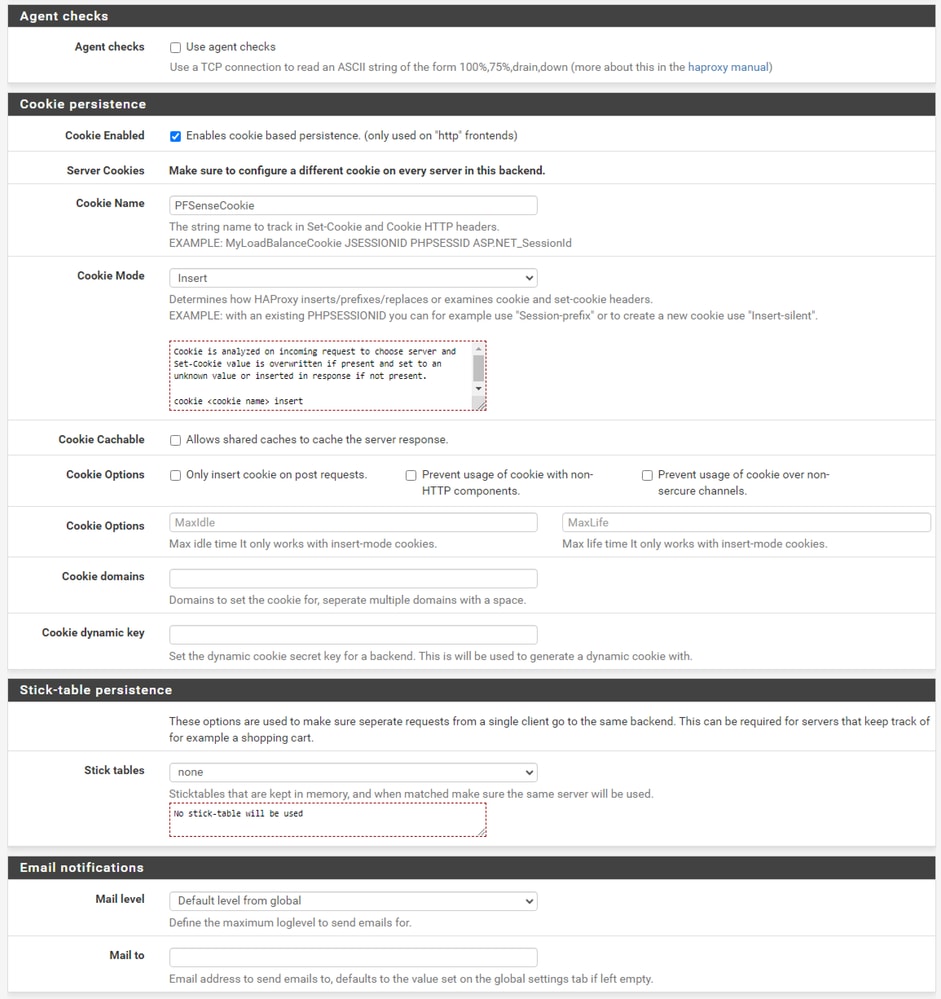The interface described contains several sections, each with different elements related to cookie settings and email notifications. Here's a detailed and clean caption:

---

The interface is organized into several distinct sections with descriptive labels and various outlined shapes containing text. 

1. **Agent Checks Section:**
   - At the top left, there's a black rectangle with the text "Agent Checks." 
   - Directly underneath, there is a white rectangle outlined in gray, also labeled "Agent Checks."
   - A gray square with text next to it is present, though the text is too small to read.

2. **Cookie Persistence Section:**
   - A black rectangle labeled "Cookie Persistence" is followed by a line of text saying "Cookie Enabled."
   - A blue square with a check mark and accompanying words, which are too small to read, sit below this.

3. **Server Cookies Section:**
   - A thin gray line separates this section, which starts with the label "Server Cookies."
   - Beneath this, illegible words are accompanied by another gray line.
   - Labeled "Cookie Names," there's a gray outlined rectangle with words inside it, followed by additional text beneath and another gray line.
   - The "Cookie Mode" label is followed by a gray outlined rectangle containing a word and an arrow pointing downward, with more text underneath.
   - A dashed gray rectangle contains unreadable text next to "Cookie Catchable."
   - Additional gray outlined squares with accompanying illegible words are present throughout.

4. **Cookie Options Section:**
   - Three gray outlined squares with words next to each are labeled "Cookie Options," followed by a gray line.
   - The label "Cookie Options" reappears with a gray outlined rectangle containing unreadable text and another identical square to the right, both with text beneath them.
   - Additional gray lines separate the elements in this section.
   - The "Cookie Domains" label outlines a gray rectangle with text underneath.
   - Further down, labeled "Cookie Dynamite Key," a gray outlined square with additional wording lies just above another gray line.

5. **Stick Table Persistence Section:**
   - A black rectangle at the bottom reads "Stick Dash Table Persistence," followed by small, hard-to-read text.
   - Another gray line leads to the "Stick Table" label, accompanied by a gray outlined rectangle containing a word and an arrow pointing downwards, with more text below.
   - An additional rectangle made of red dashed lines contains illegible words.
  
6. **Email Notifications Section:**
   - The last black rectangle says "Email Notifications," leading into text labeled "Mail Level," with a gray outlined rectangle containing words and a down arrow, followed by more unintelligible text.
   - The "Mail To" label includes a gray outlined rectangle with more text beneath it.

---

Overall, the interface features numerous sections demarcated by gray lines, black rectangles with titles, and various outlined shapes containing textual information related to cookie management and email notifications, with several portions of the text being too small to decipher.